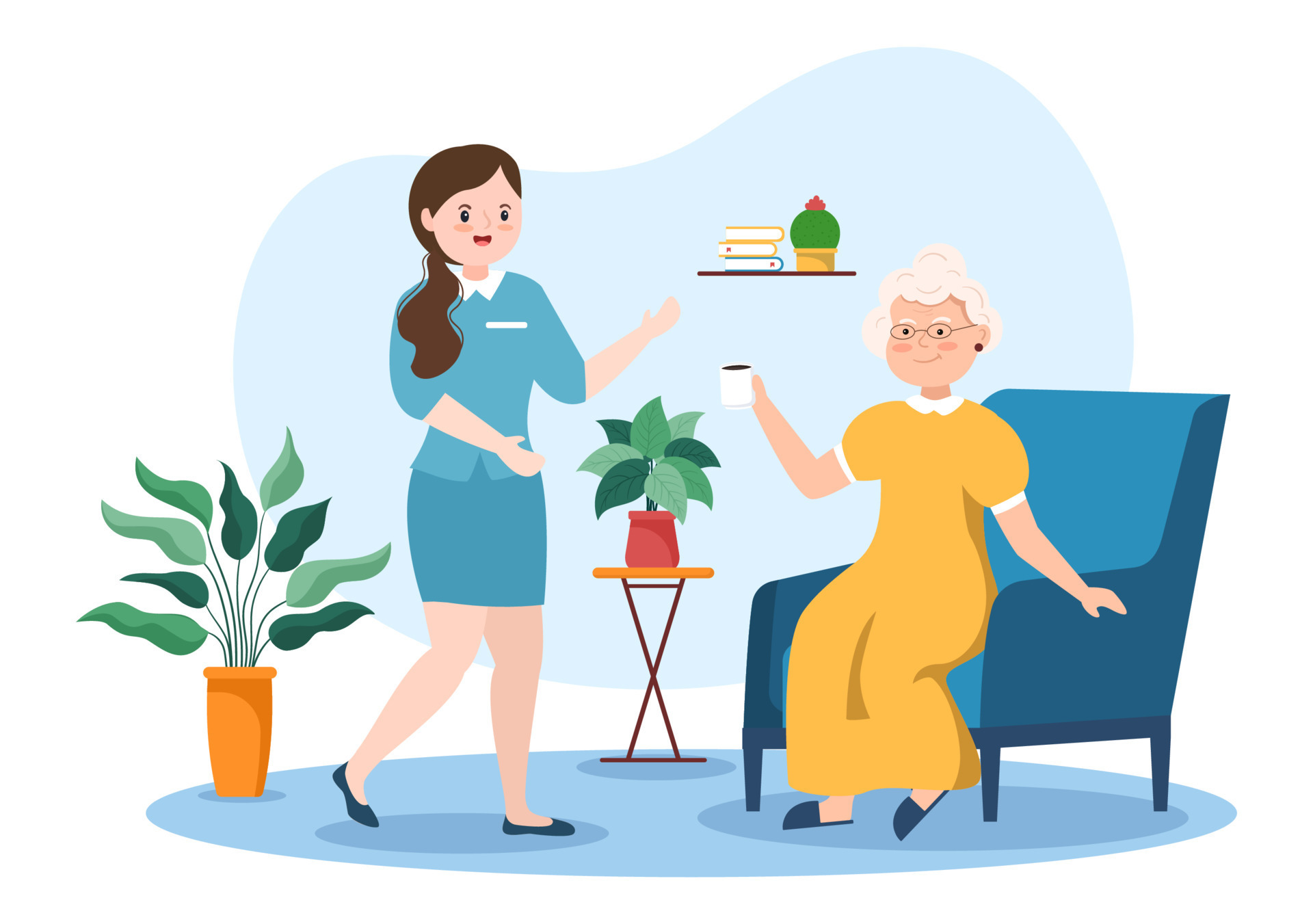This cartoonish, illustrated indoor scene features an elderly woman and a younger woman. The elderly lady, with white hair styled in a bun and round glasses, is seated on a blue armchair, wearing a long yellow dress and black slippers. She has rosy cheeks and is smiling as she lifts a coffee cup in her right hand. Adjacent to the armchair, there is a circular blue rug with a potted plant in an orange pot, featuring large green leaves that echo the shade of her dress. 

Standing nearby is a younger woman with long dark hair pulled into a ponytail cascading over her right shoulder. She is dressed in a blue blouse with a white collar and a matching short blue skirt, paired with black flats. She appears to be approaching the elderly woman, her left hand raised, possibly engaging in conversation or about to offer an embrace, smiling warmly. 

Between the two women, there is a small circular table that holds another potted plant. On the wall behind the elderly woman is a shelf containing a crown-shaped figurine and three books, along with what might be a potted cactus. The simplicity of the color scheme and the style of the illustration suggest it could be an educational graphic found in a pamphlet or PowerPoint presentation.